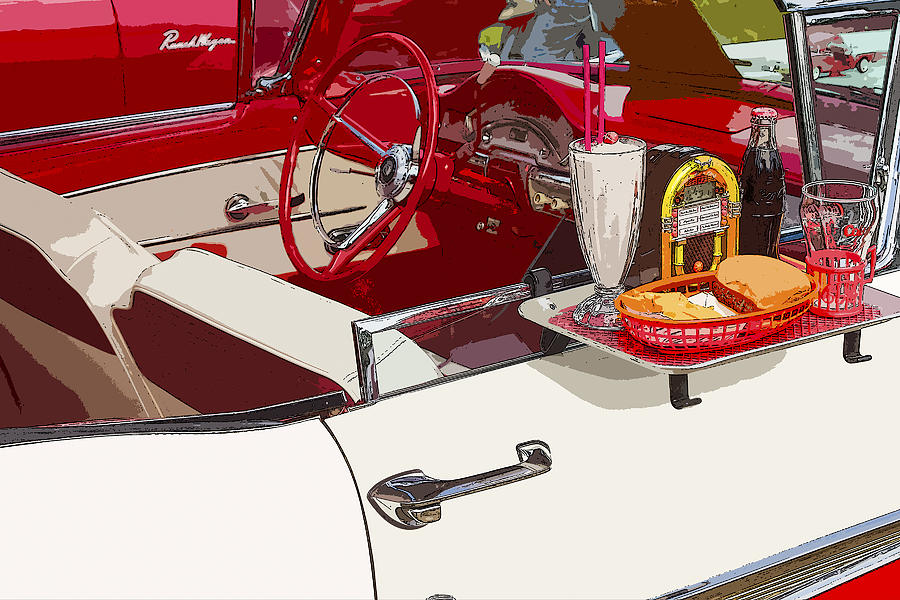The artwork is a detailed illustration of a vintage car, reminiscent of models from the 1960s or 70s, parked at a classic drive-in diner. Dominating the scene is the white car with red accents, including a candy-red steering wheel, and a mixed red and cream interior. The car's exterior showcases silver trim and chrome handles. A tray, attached to the rolled-down passenger side window, is laden with nostalgic drive-in diner items: a miniature jukebox, a white milkshake with two red straws, a glass Coca-Cola bottle, an empty clear glass, and a red basket filled with hamburgers and french fries. The angle of the artwork reveals both the passenger side and a glimpse of the driver's side, providing a view of the vintage dashboard and upholstery. In the background, partially visible in the upper left corner, is another red car, hinting at a lively, bygone era scene.